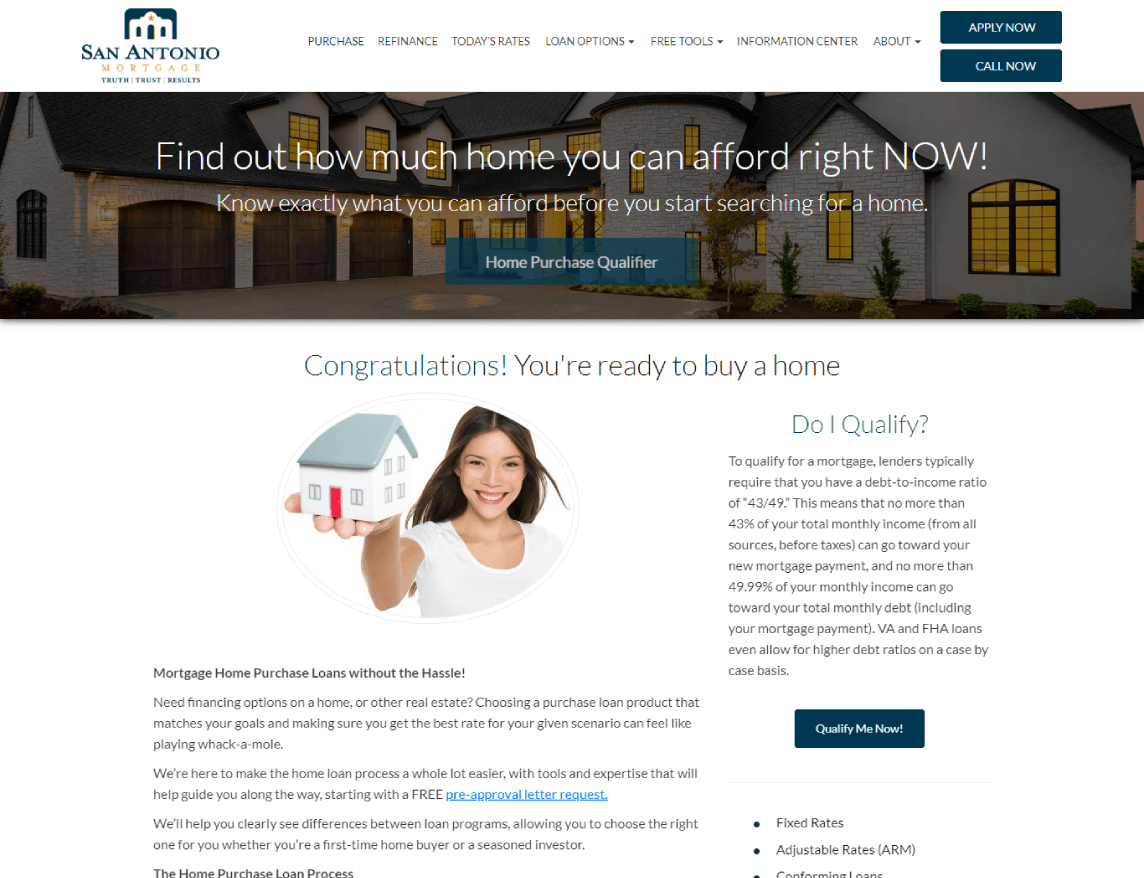This is a detailed screenshot from the San Antonio Mortgage website. In the upper left-hand corner, the logo prominently displays the text "San Antonio" beneath a stylized half-square icon that resembles a columned building. This icon includes cut-out windows on both sides and a central door. The slogan adjacent to the logo is partially legible but remains indistinct. The central portion of the screenshot features the main website menu, which includes tabs for "Purchase," "Refinance," "Today's Rates," "Loan Options" (with a dropdown menu), "Free Tools" (also with a dropdown menu), "Information Center," and "About" (with another dropdown menu). Additionally, there are prominently placed "Apply Now" and "Call Now" buttons. Below the menu is a banner featuring an image of a house and the text, "Find out how much home you can afford right now." Directly beneath this, another line reads, "Know exactly what you can afford before you start searching for a home."